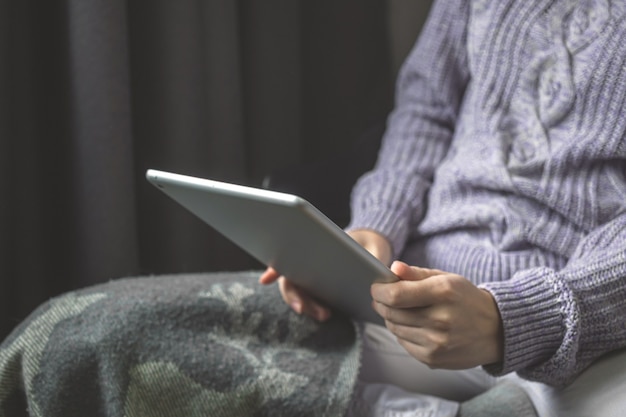In this photo, there is a woman seated and leaning slightly back, with only the lower part of her torso, hands, and knees visible as her face is out of frame. She is wearing a cable knit sweater that appears grayish-lavender in color, featuring a notable cable knit design down the center and ribbing on either side. Her hands are holding a first-generation, silver-backed iPad, with her fingers wrapped around the back and thumbs on the front. She is draped in a blanket that has white, silver, and greenish designs and is wearing white pants with her legs seemingly curled or crossed underneath the blanket. The background includes dark gray or black curtains, contributing to a cozy and somewhat chilly atmosphere, as suggested by her bundled appearance.